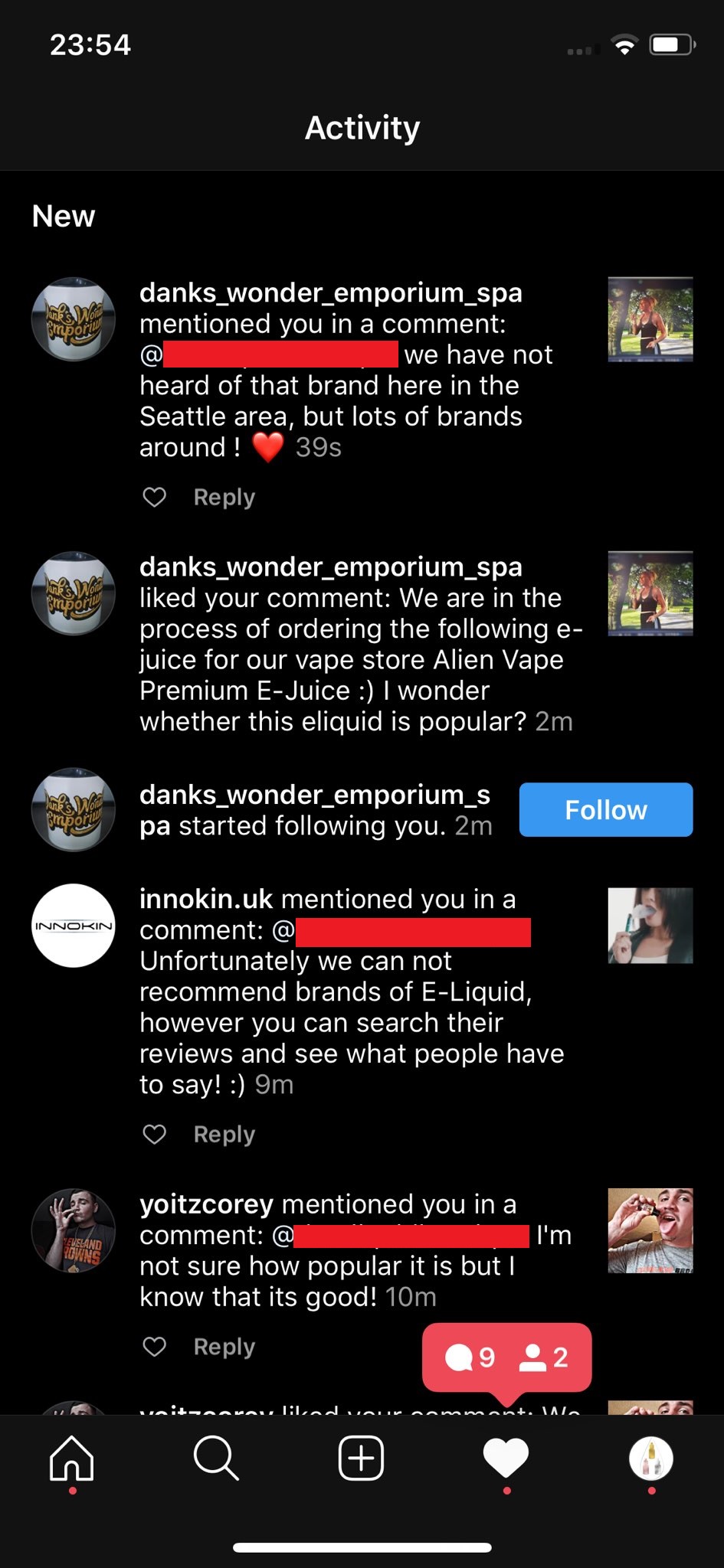A screenshot of the Instagram activity page is displayed in dark mode, featuring a dark gray background. The activity log highlights various interactions with the user's account (username censored for privacy). The recent activities include:

1. YoitzCory (Y-O-I-T-Z-C-O-R-E-Y) mentioned the user in a comment, stating, "I'm not sure how popular it is, but I know that it's good," 10 minutes ago.
2. Innokin.uk (I-N-N-O-K-I-N.U-K) responded with, "Unfortunately, we cannot recommend brands in eLiquid, however you can search their reviews and see what people have to say. :)" 90 minutes ago.
3. Danks_Wonder_Emporium_Spa started following the user two minutes ago.
4. Danks_Wonder_Emporium_Spa also liked the user's comment and mentioned them in a comment saying, "We have not heard of that brand here in the Seattle area, but lots of brands around! <3," 39 seconds ago.

This detailed activity log showcases recent interactions, including mentions, comments, likes, and new followers, all within the night mode interface of Instagram.